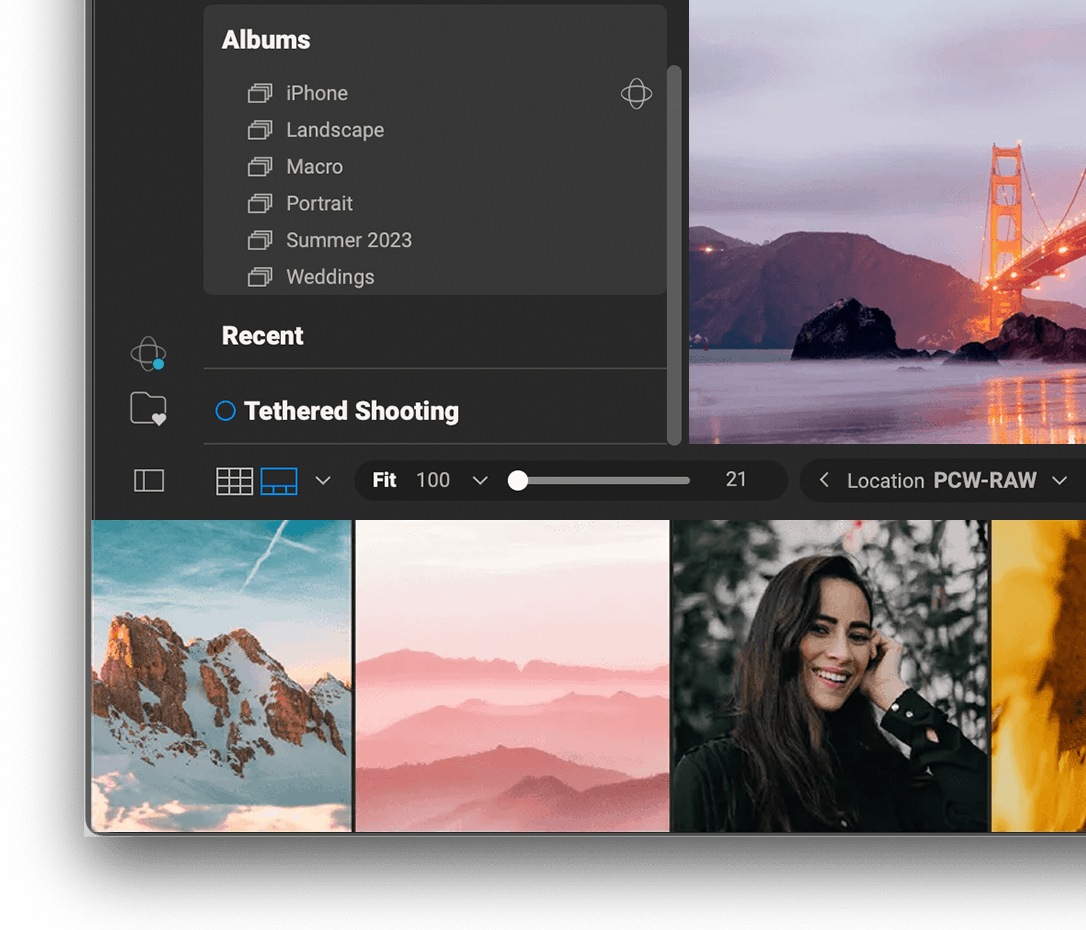The image depicts a user interface of a photo-editing website, meticulously designed for organizing and enhancing images. At the top of the interface, there's a dropdown menu labeled 'Albums,' which the user has clicked to reveal several categorizations: iPhone, Landscape, Macro, Portrait, Summer 2023, and Weddings. Each category presumably contains relevant photos.

Adjacent to the 'Albums' dropdown are icons that include a star within a blue circle, a folder with a heart symbol, and two distinct shapes—a rectangle and a square placed side by side.

Directly beneath the 'Albums' section, there are additional tabs labeled 'Recent' and 'Tethered Shooting,' though the function of the latter remains unexplained. Below these tabs, a series of symbols is visible, with one highlighted in blue, indicating it has been selected. This highlighted symbol features an adjacent dropdown menu.

Alongside, there's the term 'Fit,' followed by the number 100 with another dropdown option. Adjacent to these elements is a sliding bar, positioned fully to the left, with the number 21 displayed next to it. Further to the side, there is a label 'Location PCW-RAW' accompanied by yet another dropdown menu.

The primary workspace of the interface is filled with various images, including mountain landscapes and portraits, suggesting that the user is preparing to edit these pictures.